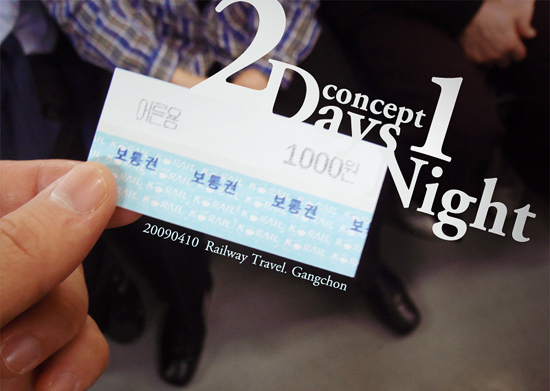This full-color photograph appears to be an ad for railway travel. Dominating the scene is a left hand holding a rectangular ticket that features a white top half with gray text and a blue bottom half with blue text in an Asian script. The numerals "20090410" and the words "Railway Travel Gangchon" can also be read on the ticket. Superimposed in large white text at the top of the image are the words "Two Days One Night Concept."

In the background, partially visible are people who appear to be standing or possibly sitting inside a train. One person is wearing a plaid shirt in yellow, blue, and white, with hands possibly folded in front of him or on his lap, and black dress shoes. Another person's well-manicured hand can be seen beside him, suggesting they too might have their hands folded. Overall, this detailed image evokes a sense of organized travel and anticipation of a scenic journey.